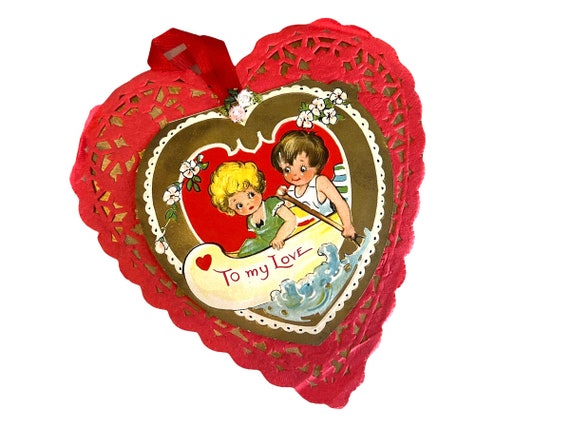The photograph captures a vintage-style Valentine's Day card set against a plain white background. The card itself is heart-shaped, crafted from red lace with a golden undertone. Intricate lace patterns create a doily-like effect with small holes. The card is slightly tilted to the left-hand side, measuring approximately 2 inches in height and width, tapering down to a fine point. 

At the very top, there is a red ribbon loop adorned with two diamond-like stones, designed for hanging. The central illustration, which has a brown border and a red background, features a little boy with black hair and a little girl with blonde hair, both of Caucasian descent, sitting in a beige canoe on blue water. The boy is rowing while they gaze at each other lovingly. A small red heart is visible on one side of the canoe, beside red text that reads, "To My Love." Surrounding the red heart in the center are delicate white flowers, adding a charming touch to the nostalgic design.